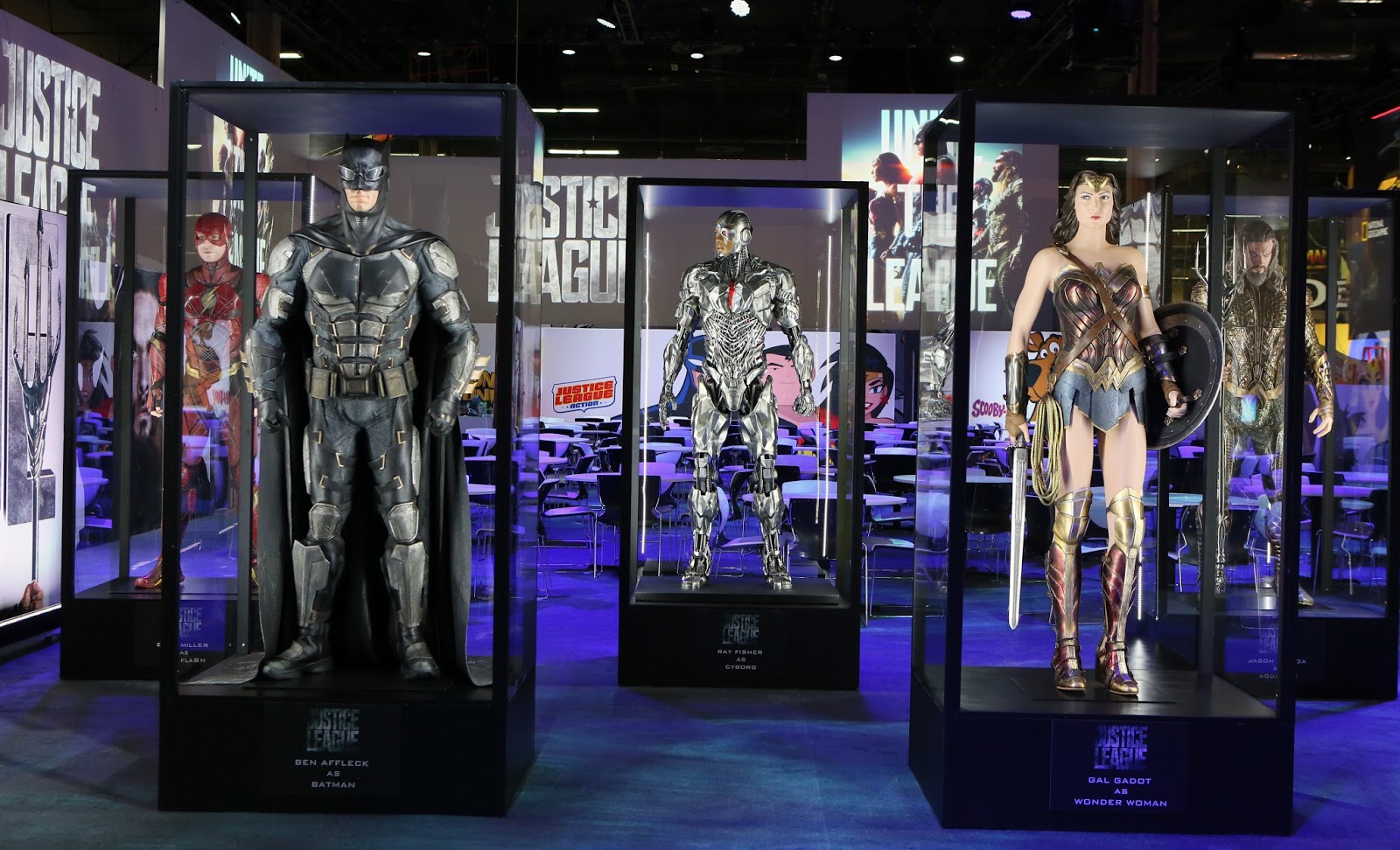The photograph showcases an elaborate display at a convention or museum dedicated to Hollywood costumes from the Justice League. Central to the exhibit are five encased glass enclosures, staged with mannequins adorned in detailed, lifelike replica costumes from the Justice League movies. Arranged from left to right, the characters are The Flash in his signature red suit, Batman, Cyborg, Wonder Woman clad in her iconic armor, and Aquaman. Each glass case, set on a sleek black base, has placards identifying the actors: "Justice League, Ben Affleck as Batman," "Justice League, Ray Fisher as Cyborg," and "Justice League, Gal Gadot as Wonder Woman." The background is adorned with various Justice League imagery from both recent films and classic cartoons. The cases are well-lit, allowing for clear visibility of the intricately designed costumes. Beyond the displays, the setting includes tables and chairs, suggesting an open, possibly multipurpose space.